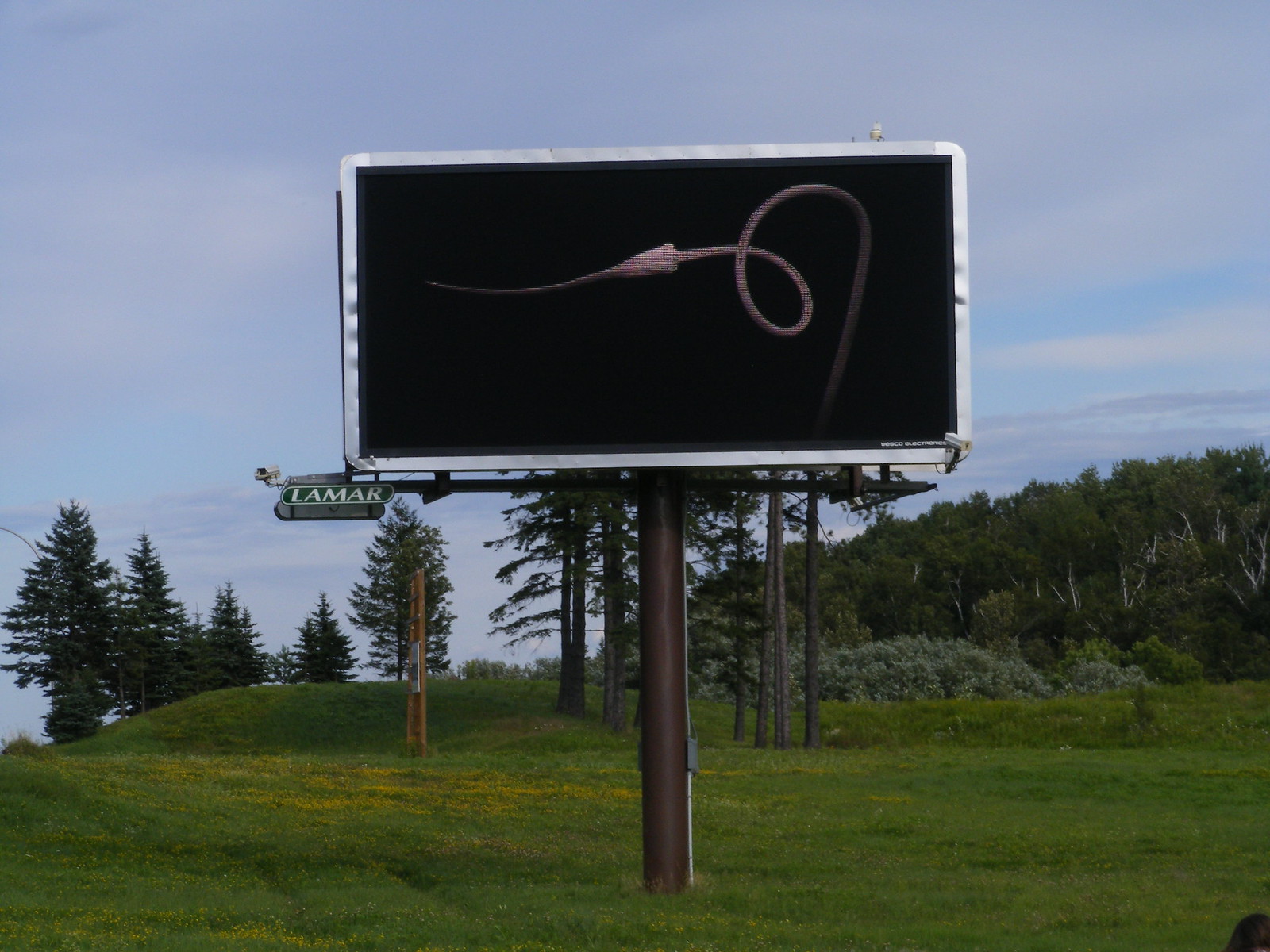The photograph captures a scenic countryside setting in America. Dominated by lush, green grass with a few yellow patches, the landscape features rolling grassy mounds and a cluster of trees, including tall evergreen firs and trees with white trunks and green leaves. A striking blue sky with thin white clouds forms the backdrop. Central to the image is a freestanding digital billboard mounted on a tall, solid brown post with a white border. The billboard, owned by Lamar—as indicated by their logo in a brown rectangle on the lower left—displays a black screen with a peculiar image resembling a cross between a worm, a magic mushroom, and possibly a sperm. Laminated with silver edges, this high-tech sign is flanked by security cameras on both ends, adding an element of surveillance to the serene rural scene.